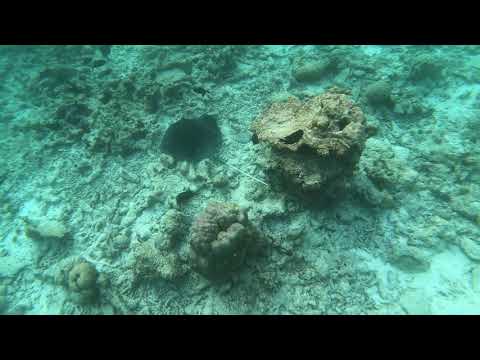This underwater photograph, taken in the clear, pale green waters at the bottom of the ocean, captures a scene teeming with marine life and diverse coral structures. Dominating the center of the image are two large pieces of coral with differing species amidst an irregular ocean floor. Between these corals and toward the left upper quadrant of the picture, a black stingray with a long white tail gracefully glides. The seabed is scattered with rocks of various shapes and sizes, primarily in brown, white, and gray colors, creating a contrasting mosaic against the predominantly green and turquoise backdrop. To the right, a small gray rock-like formation stands out, while to its left, a hole can be seen. Above this hole, different types of sea plants appear, adding to the rich biodiversity depicted in this vibrant underwater scene.